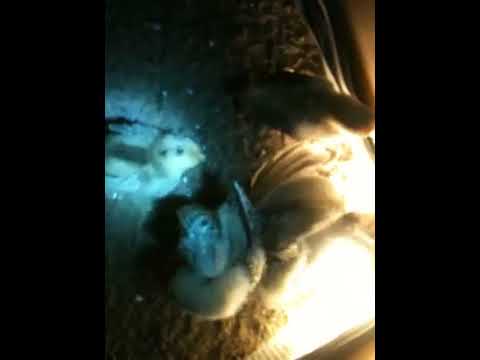The image features a central composition with a variety of indistinct objects, predominantly centered, and obscured by the complex interplay of colors, including white, yellow, brown, light blue, black, and tan. The image is bordered by thick black bands on both the left and right sides, framing the main content. Notably, the upper right portion of the image displays what appears to be the head of an animal, potentially a cat, facing left with an ear extending to the right. This animal is draped in what seems to be a blanket spread across its body. Adjacent to this animal head, towards the left, there are ambiguous items that might be toys or slippers, with one resembling a duck facing right, identifiable by its small beak and eye. The bright bottom right corner suggests reflected light, contrasting with the darker upper regions. The detailed textures and subtle glowing specks scattered throughout contribute to a somewhat grainy quality, making it challenging to clearly identify the objects or the setting depicted in the photograph.